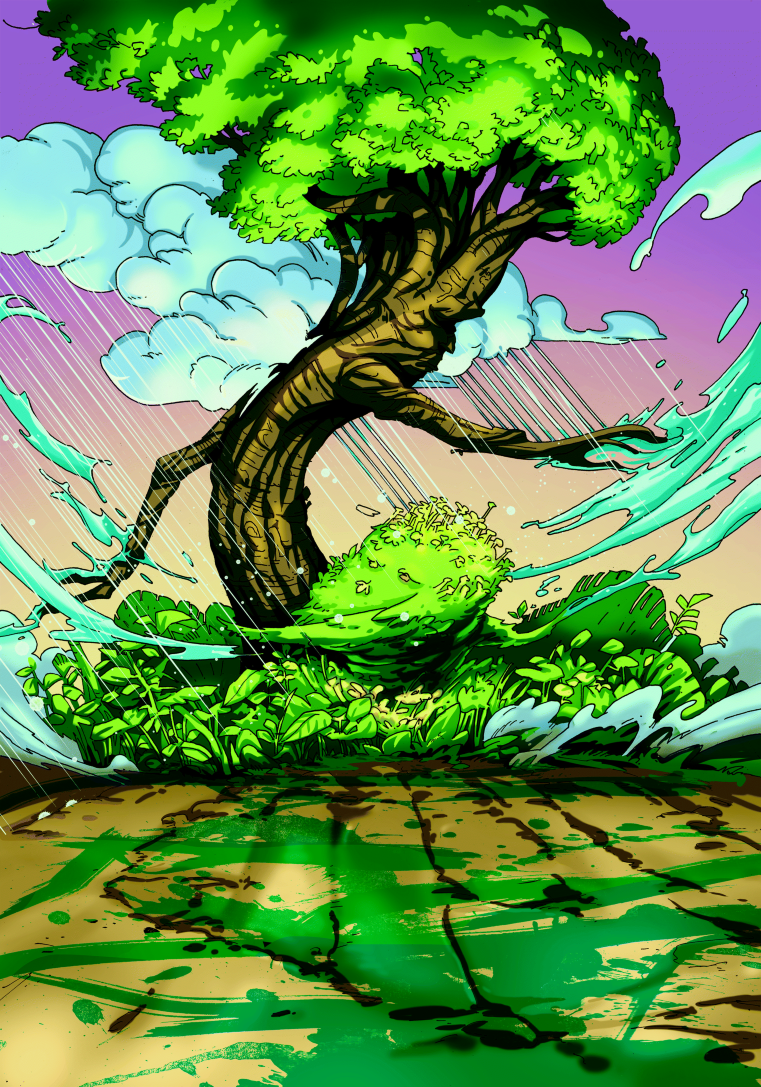This detailed digital image, reminiscent of Japanese art, features a prominent tree with brown bark and various shades of green in its cartoonish leaves. The image is in portrait layout, depicting a tree leaning slightly forward as if caught in a gust of wind. Surrounding the tree is a dramatic sky filled with hues of purple, pink, and orange, seamlessly blending into a light peach color. White and bluish clouds scatter across the sky, contributing to the impression of an ongoing windstorm or rainstorm. Sheets of rain appear to be descending from the clouds, with visible streaks and splashes of water hitting the ground on both sides of the tree. At the tree’s base, there is an array of green foliage and leaf plants, characterized by their almost trapezoidal shapes pointing in various directions.

The ground in the image consists of a brownish-yellowish-cream color, possibly representing dirt, with patches reminiscent of green paint splatters, suggesting grass. The lower third of the image includes a distinct light brown path, reminiscent of a large Japanese symbol. This path leads up to a bush with yellow flowers at the center. Notably, the trunk of the tree features indentations that resemble eyes, a nose, and a mouth, giving it a humanoid appearance. Branches extend from this anthropomorphic trunk, with limbs stretching out to touch descending sheets of water. Together, these elements create a vivid, dynamic scene capturing the essence of an intense weather event intertwined with artistic whimsy.